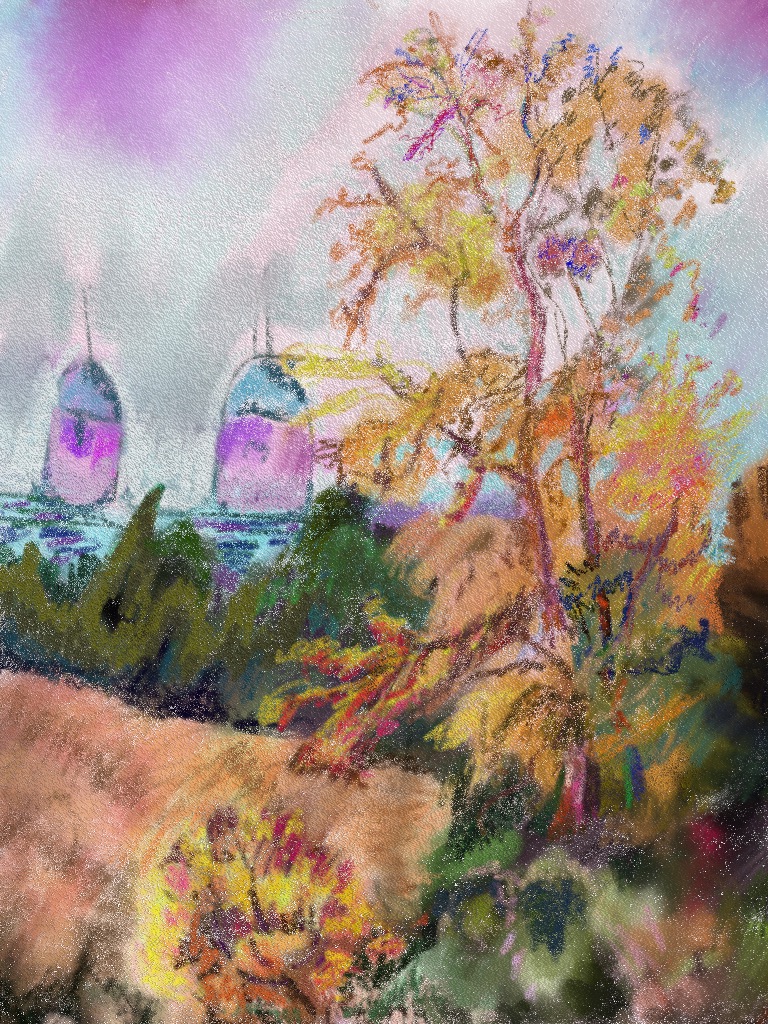This image showcases a beautiful painting that appears to be created using a medium other than watercolor, possibly oil paint or a similar artistic medium, characterized by its streaky and fluid appearance. The composition depicts a serene shoreline scene adorned with vibrant autumnal trees bearing orange leaves and a small bush also sporting orange foliage. A prominent sandy, or perhaps yellow-tan, area stretches across the foreground, adding contrast to the lush, albeit somewhat indistinct, vegetation that appears somewhat blob-like in form.

In the far background, the vast expanse of the ocean meets the horizon line, complemented by a purplish-blue sky that envelops the scene in a calm, twilight ambiance. Upon closer inspection, two ships can be seen far out in the ocean, distinguished by their unique purple hulls, adding a dash of intrigue and distant activity to the otherwise tranquil landscape. The overall effect is a picturesque and slightly abstract representation of nature's beauty, captured through the artist’s unique style and choice of medium.